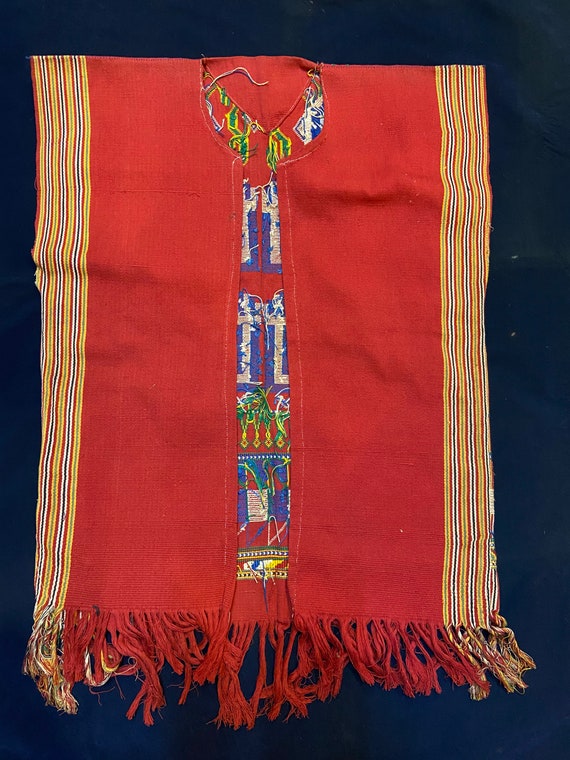This image features a vibrant, sleeveless cultural garment that resembles a poncho or vest, set against a black background. The material appears to be of rough, textured cloth in a predominant dark orange-red hue. Both sides of the garment are adorned with vertical yellow and orange stripes, complemented by additional white stripes, suggesting a traditional textile display. The neckline is richly decorated with a multicolored patchwork containing green, yellow, blue, and white elements, possibly representing significant cultural symbols or achievements. The central section of the garment, where buttons might traditionally be placed, features intricate blue and white patterns, alongside green and yellow motifs that could be depicting forestry or figures, possibly a person riding a horse. Adding to its elaborate design, the bottom of the garment has a fringe, continuing the orange, yellow, and white color scheme, reminiscent of the ends of a woven rug. The interior also showcases complex patterns in blue and green, enhancing its detailed appearance.